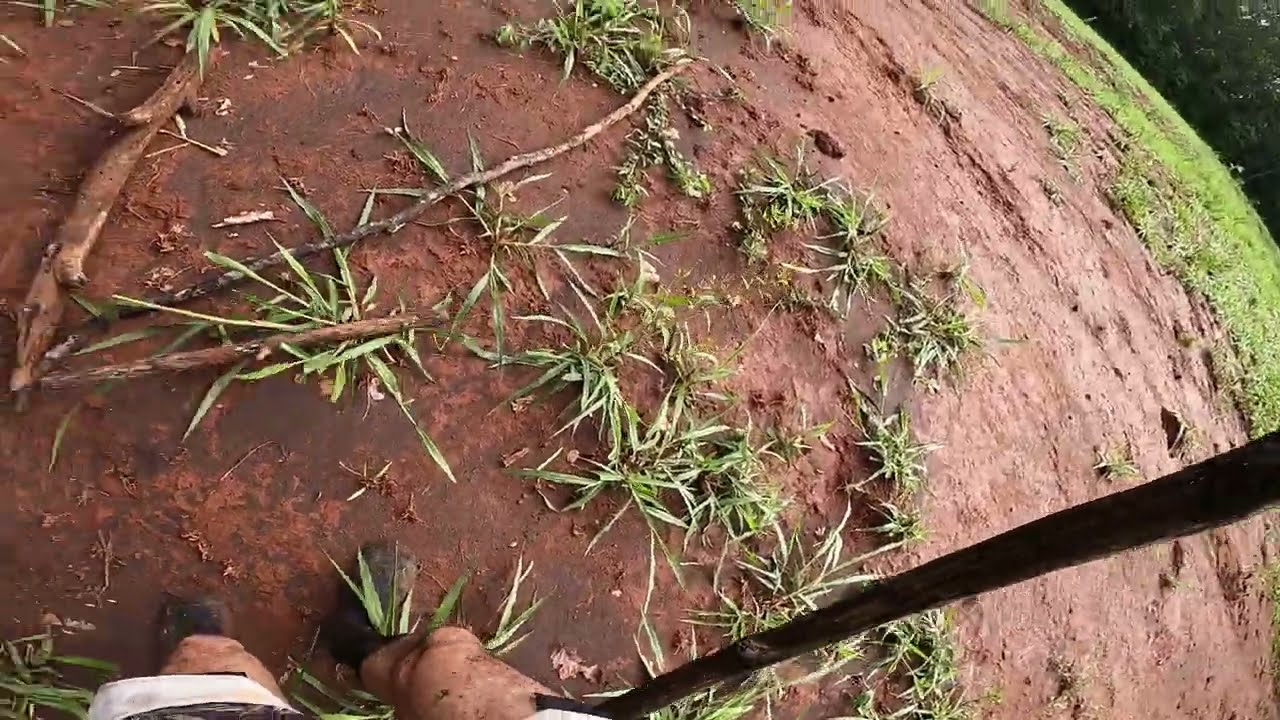The photograph captures a scene where a person, possibly the photographer, is standing in a muddy, reddish-brown, clay-like ground. The ground is wet and predominantly composed of this clay-mud mixture, with patches of sparse grass particularly visible towards the left side of the image. The person, who appears to be a man, is wearing black boots and white shorts that expose much of his legs, which appear dirty from the mud. He is holding a stick or makeshift cane against his bare leg. Scattered around are some brown wooden sticks or branches. In the background, the image reveals a small portion of trees, though they are not the central focus of the photograph. The lighting suggests a diffused, overcast sky, contributing to the lack of harsh shadows and implying it might be cloudy. The overall setting gives the impression of a muddy, possibly jungle-like area, with the person seemingly engaged in an activity that involves navigating or wading through the mud.